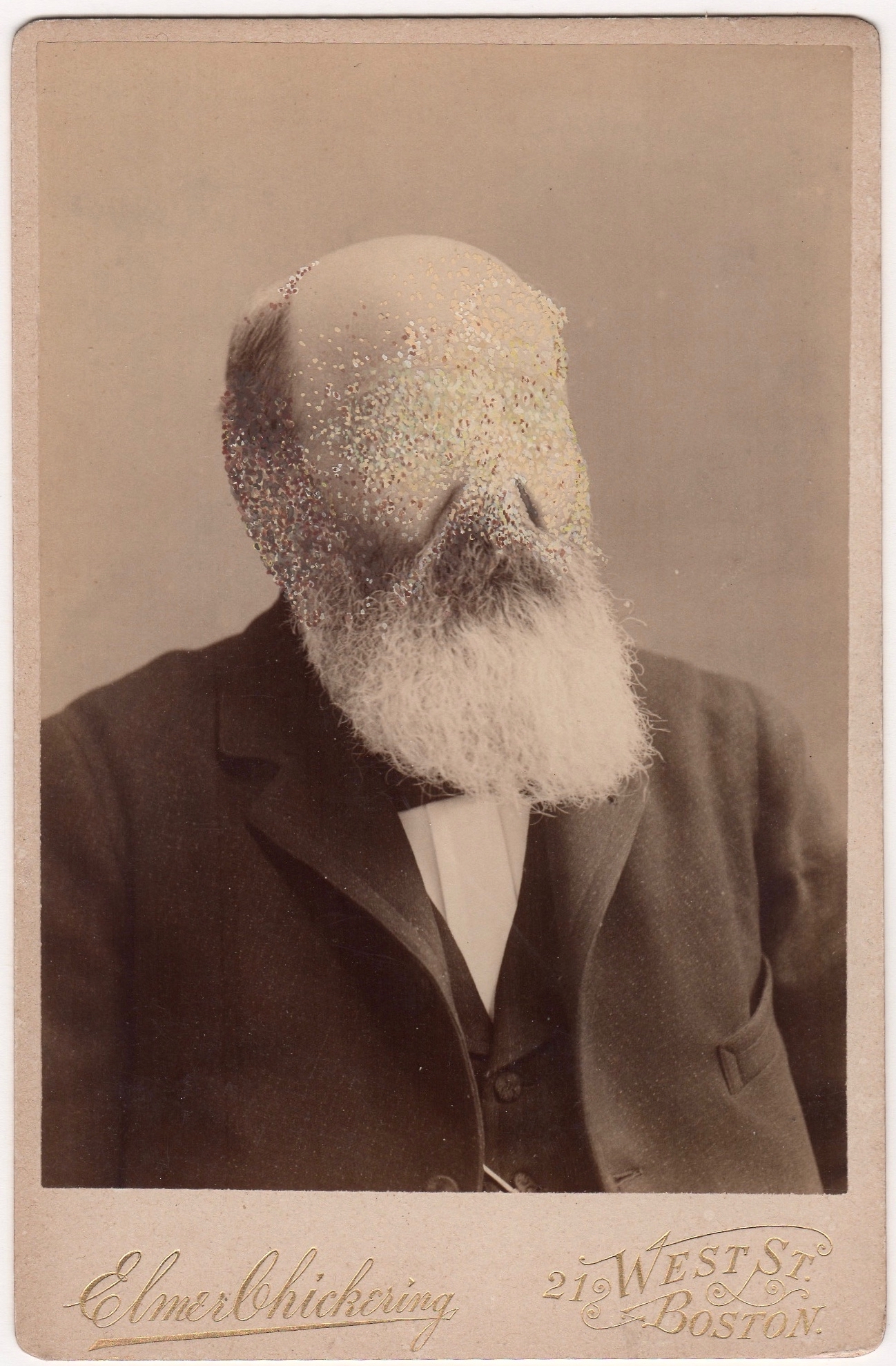In this eerie, deteriorated black-and-white photograph, a balding man with a prominent white beard and a dark mustache is depicted, dressed in a formal suit comprising a blazer, a bow tie, a vest, and a crisp white shirt. Strikingly, his eyes, nose, ears, and eyebrows are missing or obscured, leaving only his beard and some patches of dark hair visible. The image quality appears damaged, with sections that seem rubbed off or disintegrating, creating a speckled, ghostly effect, particularly on his facial features. The haunting nature of this tall, rectangular photograph is enhanced by its weathered state, suggesting significant age. At the bottom of the image, in elegant cursive script, the name "Elmer Chickering" is inscribed, followed by "21 West Street, Boston," likely indicating the photographer's studio or the location where this enigmatic portrait was captured.